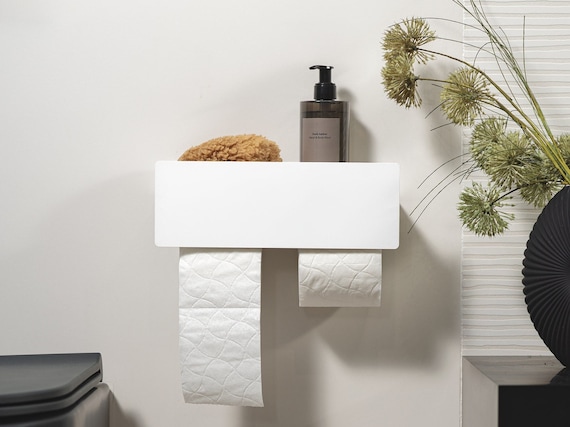This photograph captures a modern bathroom setup, centered around a sleek white shelving unit that dispenses two rolls of toilet paper. The roll on the left has several sheets hanging down, while the roll on the right remains intact. Resting on top of the dispenser are a black soap container and a sponge, alongside what appears to be a loofah and possibly some lotion. The bathroom's white wall backdrop enhances its minimalist aesthetic. To the right of the dispenser, white slat window blinds are partially visible, accompanied by a black vase containing green and white flowers, adding a touch of vibrancy. The left side of the image hints at either a trash can or a laundry basket with a black top, partially off-screen. The overall atmosphere of the bathroom is modern and somewhat cold, evoking a museum-like cleanliness.